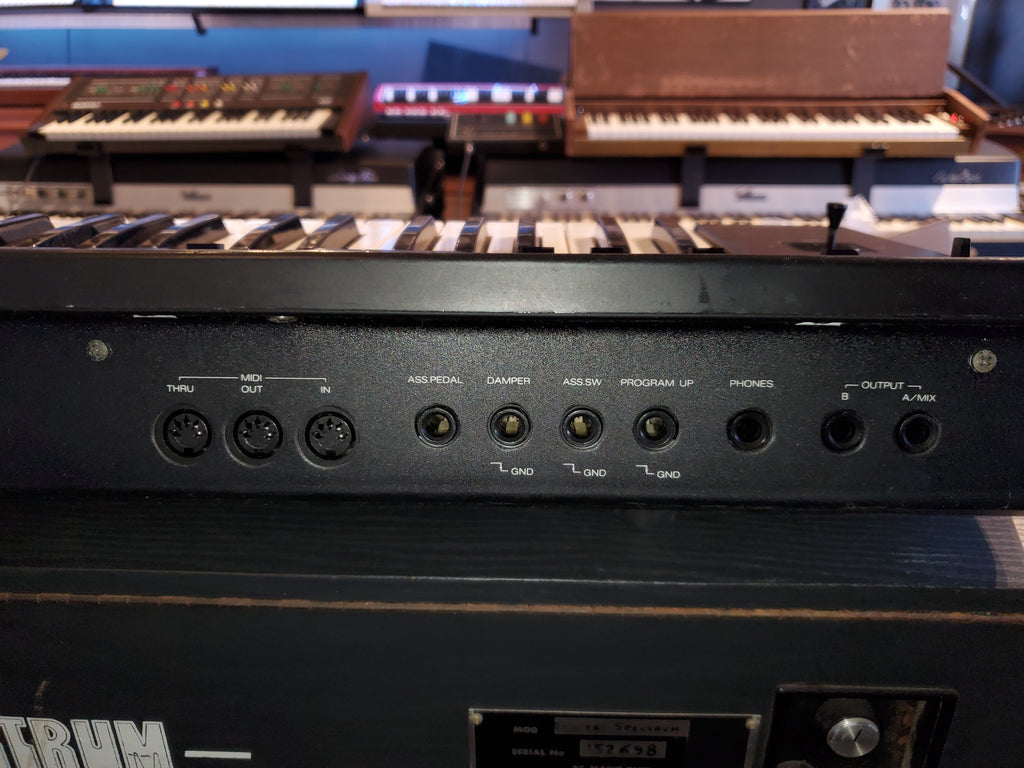The image features a detailed view of the back panel of an electronic keyboard. The instrument itself is black, with various ports and jacks labeled for connectivity, including MIDI in, out, and through, as well as jacks marked for input, output, and headphones. Notably, there are also sections labeled ASSW, program up, and a switch likely for volume control. The keyboard is positioned upright on a black platform. 

In the background, a variety of other keyboards and musical equipment are visible, including a brown Casio keyboard with black, white, and some red and yellow keys and buttons. Positioned nearby is a piano encased in wood, with standard black and white keys, and another blue electronic device, though it's partially out of focus in the image. The overall scene appears to be set in a studio or a musical workspace filled with an array of electronic and traditional keyboards.